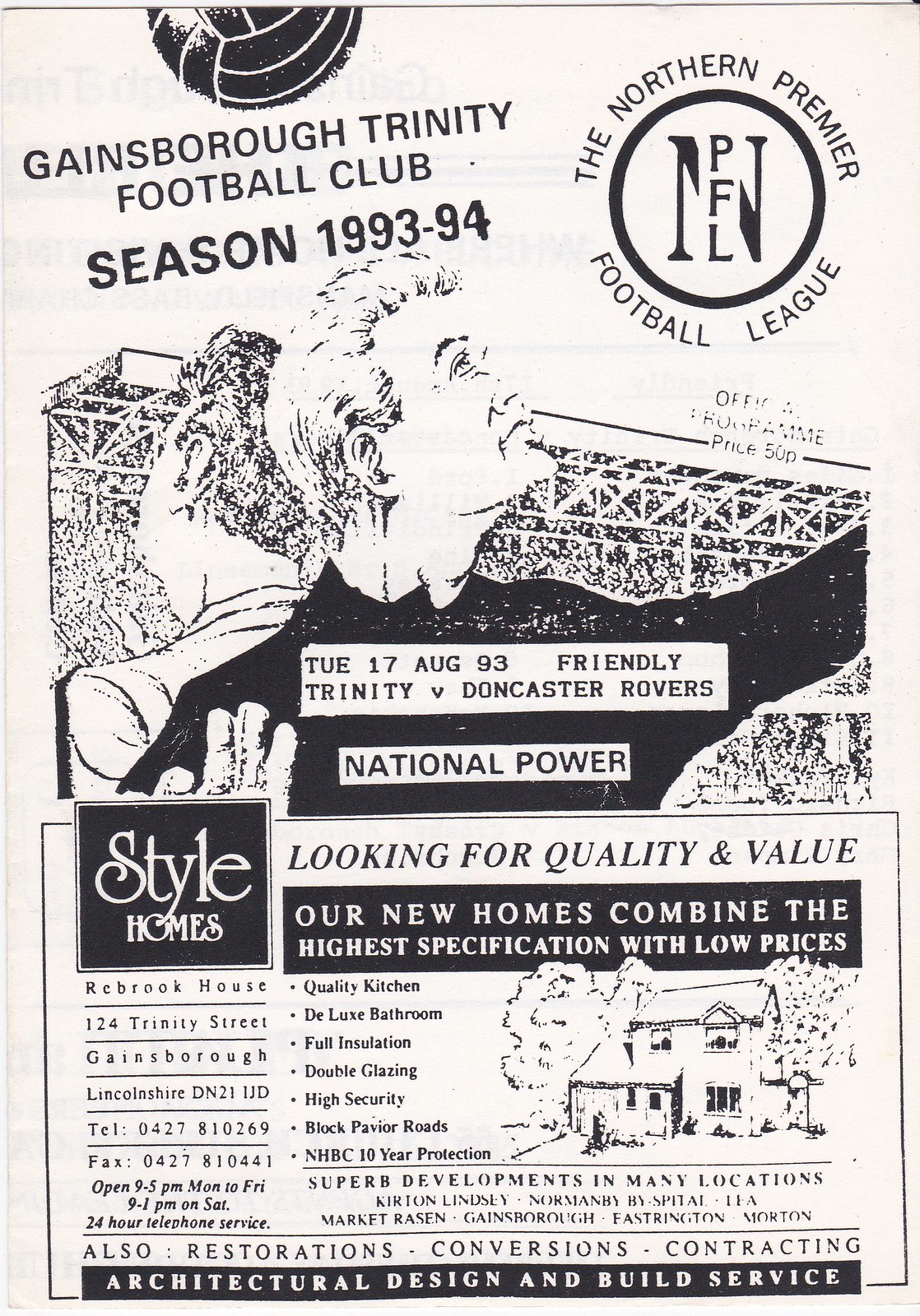This black-and-white advertisement or flyer is for the Gainsborough Trinity Football Club's 1993-94 season. The top left corner prominently features "Gainsborough Trinity Football Club Season 1993 to 94," while the top right showcases the Northern Premier Football League logo. Below this, the date "Tuesday 17th August 93" is highlighted, indicating a friendly match between Trinity and Doncaster Rovers, noted as a national power.

The central image is a pencil sketch of two male fans standing back-to-back, appearing to be in front of bleachers or stands. The man in the foreground extends his arm upward. Below this scene, there's a detailed advertisement for Style Homes, promising quality and value with features like quality kitchens, deluxe bathrooms, full insulation, double glazing, high security, and HBC 10-year protection. The ad also mentions the development of superb locations, including Gainsborough and Market Rasen, although the latter is hard to decipher.

Style Homes is located at Rebrook House, 124 Trinity Street, Gainsborough, Lincolnshire, DN21, IJD. The advertisement includes contact details: telephone 0427 810269, fax 0427 810441, and specifies opening hours from 9 to 5 Monday to Friday, and 9 to 1 p.m. on Saturday, with a 24-hour telephone service. Along the bottom of the ad, services such as restorations, conversions, contracting, architectural design, and build services are also mentioned.